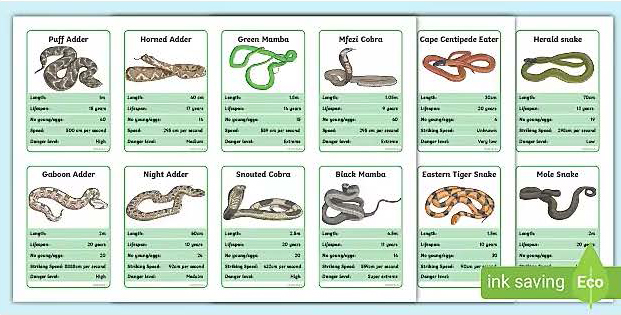This image is a detailed chart featuring 12 different types of snakes arranged in two rows on a light blue background. Each snake is presented on a rectangular card that includes a name in black text at the top, an illustration of the snake occupying the upper half of the card, and a green section at the bottom that contains various statistics in small, hard-to-read text. The snakes are arranged in the following order from left to right: the first row includes the Puff Adder, Horned Adder, Green Mamba, Mefzi Cobra, Cape Centipede Eater, and Herald Snake; the second row has the Gaboon Adder, Night Adder, Snouted Cobra, Black Mamba, Eastern Tiger Snake, and Mole Snake. The Puff Adder and Horned Adder have brown patterned scales, while the Green Mamba is solid green. The Mefzi Cobra features light brown coloration with dark spots and a distinctive head, the Cape Centipede Eater is red with a black head, and the Herald Snake is dark green. In the bottom row, the Gaboon and Night Adders are brown with spots, the Snouted Cobra has a light brown or green body with distinctive dark spots, the Black Mamba is dark gray, the Eastern Tiger Snake is orange with black bands, and the Mole Snake is dark gray or green. In the bottom right corner is a green rectangular logo that says "Ink Saving Eco" in white text, accompanied by a leaf image beneath the word "Eco."